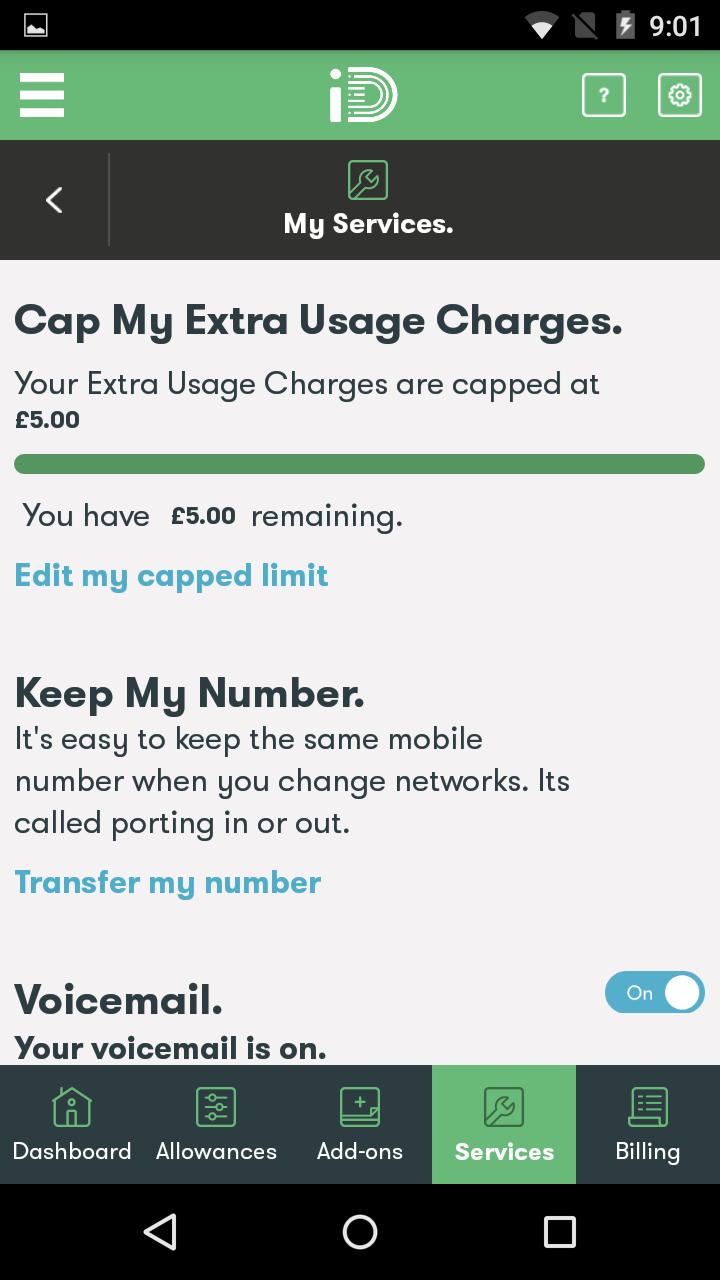This mobile screenshot features a detailed interface with multiple icons and headers. At the top, there is a black header bar with a white image icon resembling a bordered square with a mountain inside. To the right of this icon, a WiFi signal indicator displays two-thirds strength, followed by a gray 'no SIM' icon. Further to the right, a gray battery icon with a white lightning bolt signifies that the device is charging. The white digital clock on the far right reads "9:01."

Below the black header, a section with a light mossy green background appears. On the left side of this header, there are three bold white lines representing a dropdown menu. Centrally located is a logo design featuring a bold lowercase "i" and a partially completed "D" with a thick outline on the top, bottom, and right, transitioning into several horizontal lines. To the right of the logo, a white square outline with a question mark in the center indicates a help option. Further right, a white gear icon enclosed in a white box represents settings.

Directly underneath, an off-white header includes a white arrow pointing left on the left side, followed by a very faint gray dividing line. Centered in this section, a green square with a wrench icon represents tools, accompanied by bold white text reading "My Services."

Further down, a section with a light gray background and black bold text at the top left reads "Cap My Extra Usage Charges." Below this, smaller, non-bold black text states, "Your extra usage charges are capped at" followed by a bold black "£5.00."

This detailed interface provides users with clear navigation options, status indicators, and capped limit information, all within a visually cohesive design.